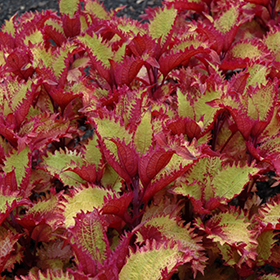The photograph captures a close-up of a mass of striking and uniquely beautiful plants, possibly Venus flytraps or another type of carnivorous plant like coleus. The image, taken outdoors with some shading, showcases clusters of leaves that crowd tightly together, revealing intricate details. Each leaf has a vibrant lime green interior framed by a deep rose or magenta border, giving the impression of tiny flames. The spiky or ruffled edges add to the textured appearance of the leaves. While the leaves' undersides are a darker reddish-pink, the upper surfaces display a blend of yellowish-green hues. The background partially shows bits of brownish-gray, possibly mulch, adding a natural frame to the densely packed, colorful foliage.